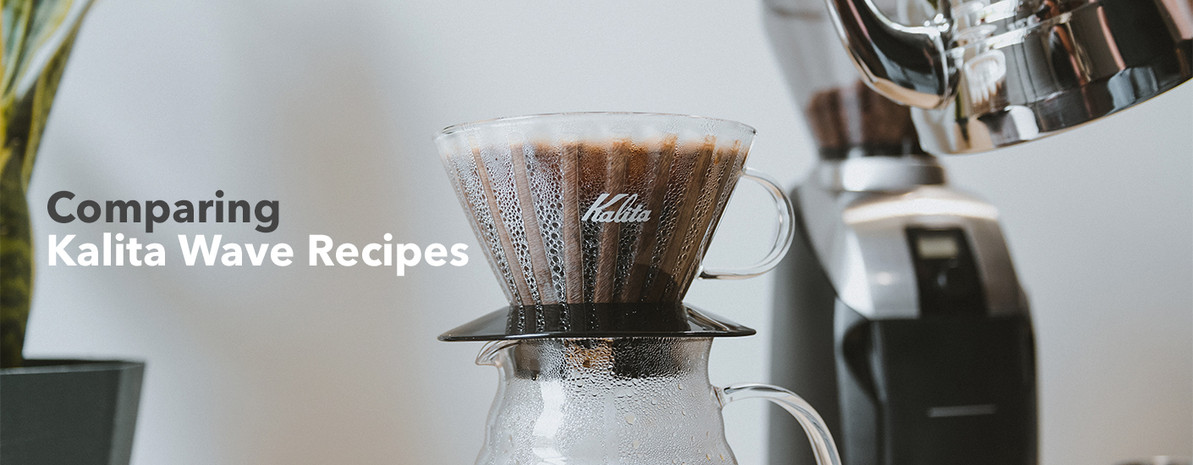The image shows a close-up display of a clear coffee cup, prominently featuring the word "Kalita" in white letters on its side. The cup, with a black circular base, sits atop a glass pitcher that has visible moisture droplets on its surface, indicating condensation. The arrangement is part of a professional coffee setup, with the photograph likely illustrating a comparison of Kalita Wave recipes, as suggested by the text "Comparing Kalita Wave Recipes" on the left side. The background displays additional coffee equipment, including a silver object resembling the base of a coffee or tea cup on the right, and a coffee grinder with a black base, gray section, and plastic beans container at the top. The backdrop is dominated by varying shades of gray, complemented by the brown liquid inside the cup and the green leaves of a plant in a pot on the far left. Overall, the setup has a clean, professional aesthetic, with an emphasis on coffee brewing.